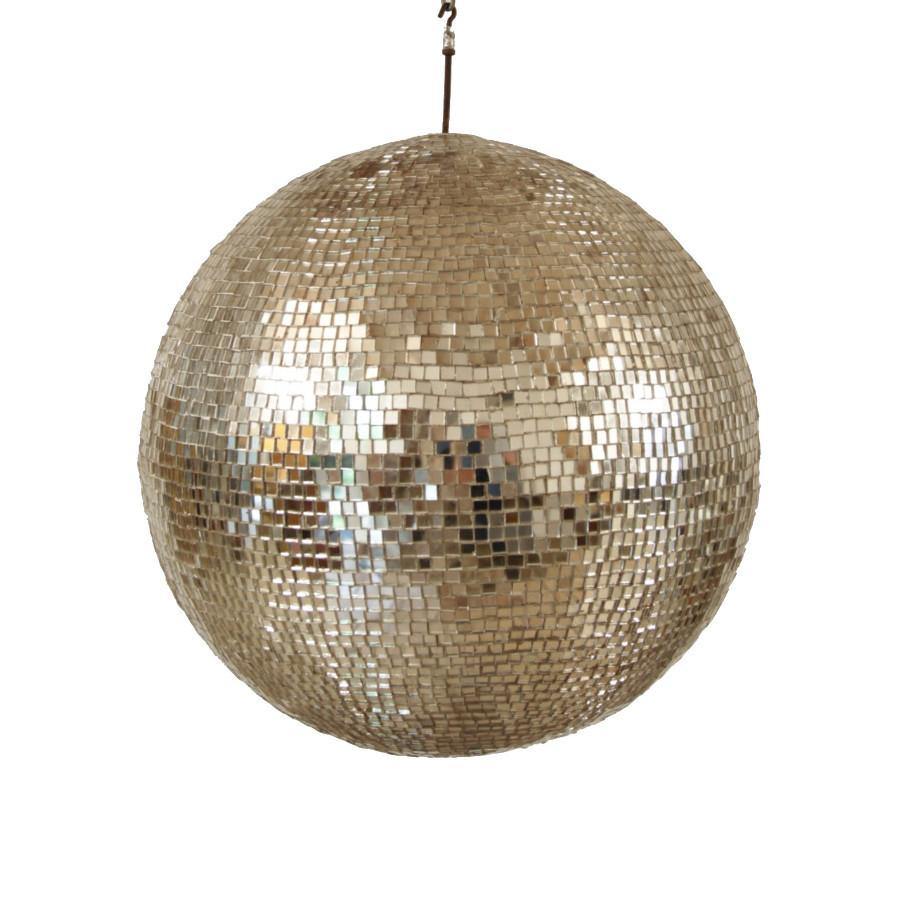A glittering ornament hangs prominently, its reflective surface catching and dispersing light in a kaleidoscope of hues. Attached by a thin string with a small hook, it suggests a potential use as a festive decoration, likely for a Christmas tree. The ornament resembles a miniature disco ball, comprised of hundreds of tiny, square tiles arranged meticulously across its spherical surface. The majority of these tiles feature a muted gray-moth coloration, although light striking different angles causes variations—some sections appear white, tan, black, or darker shades of gray. The top and front-middle of the ornament are less illuminated, casting subtle shadows that lend depth to its textured appearance. The play of light and shadow, combined with the mosaic of reflective tiles, creates a visually captivating object that evokes the charm and sparkle of the holiday season.